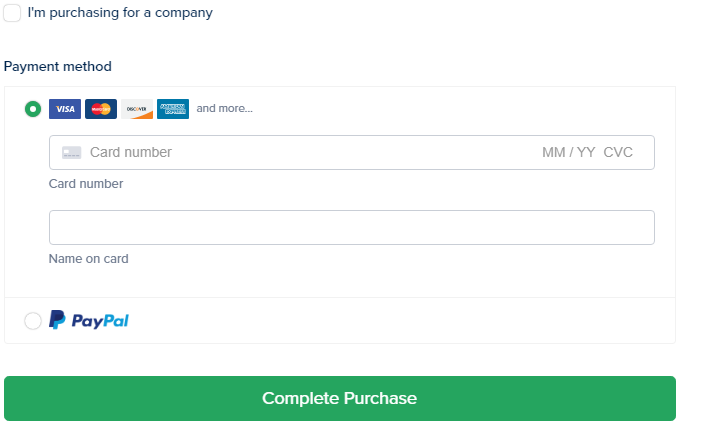The image is a screenshot of a payment page on a website, featuring a clean, white background with various form elements and a green bar at the bottom. In the upper-left corner, there's a clickable checkbox labeled "I'm purchasing for a company." Below that is a section titled "Payment Method," where the user has selected the credit card option indicated by a small green circle.

Adjacent to this, there's a row displaying different credit card icons such as Visa, MasterCard, Discover, and American Express, with a note indicating "and more." Below this row is a large, horizontal gray box labeled "Card Number," with fields for "MM/YY" and "CVC." Another horizontal box beneath this is labeled "Name on Card."

Further down, there's an option to select PayPal as a payment method, represented by an empty circle, indicating it was not chosen. Dominating the bottom portion of the image, a large green bar spans from left to right. In the center of the bar, white text boldly states "Complete Purchase." 

Overall, this screenshot captures the elements of a web page designed for completing a financial transaction.